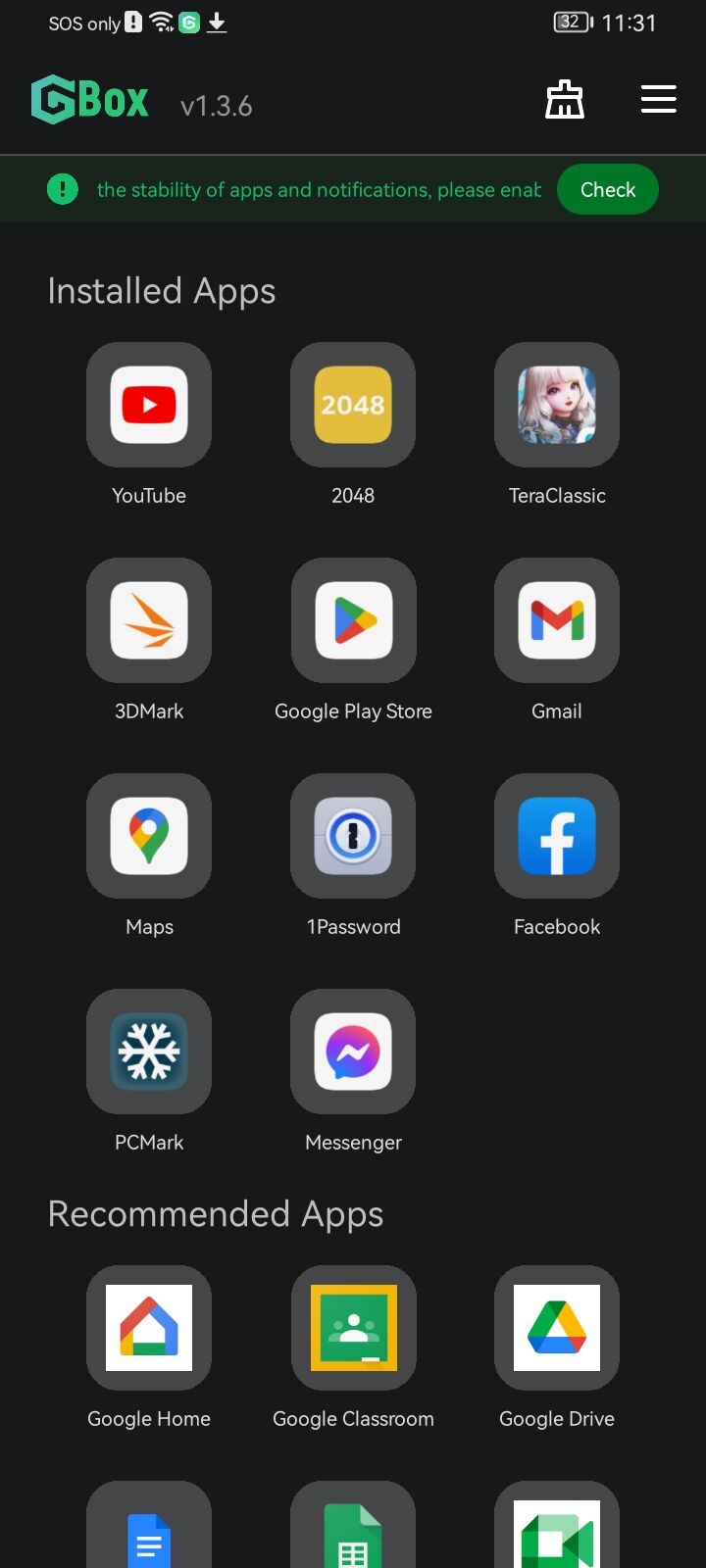The image depicts the screen of a cell phone with several details visible. At the very top of the screen, the status bar indicates "SOS only" for network connectivity, a Wi-Fi icon, a download notification, a battery level at 32%, and the time reading 11:31. On the top left corner, there's a green icon labeled "GBOX" with the version number "V1.3.6." On the top right corner, three horizontal lines can be seen, along with an unidentified icon.

Below the status bar, there is a notification banner with a green background overlaid with black. The banner features an exclamation point inside a circle and a partially displayed message that reads "The stability of apps and notifications, please E-N-A..." followed by a "Check" button.

The screen then lists "Installed apps" including YouTube, 2048, TerraClassic, Gmail, Google Play Store, 3DMark, Google Maps, 1Password, Facebook, Messenger, and PCMark. Following this, under "Recommended apps," Google Home, Google Classroom, and Google Drive are displayed, along with icons for Google Docs, Google Sheets, and an unidentified app.

All icons are set against a black background, with each button featuring a gray base, an app-specific icon on top, and white text. The colors of the icons predominantly include red, yellow, and green.